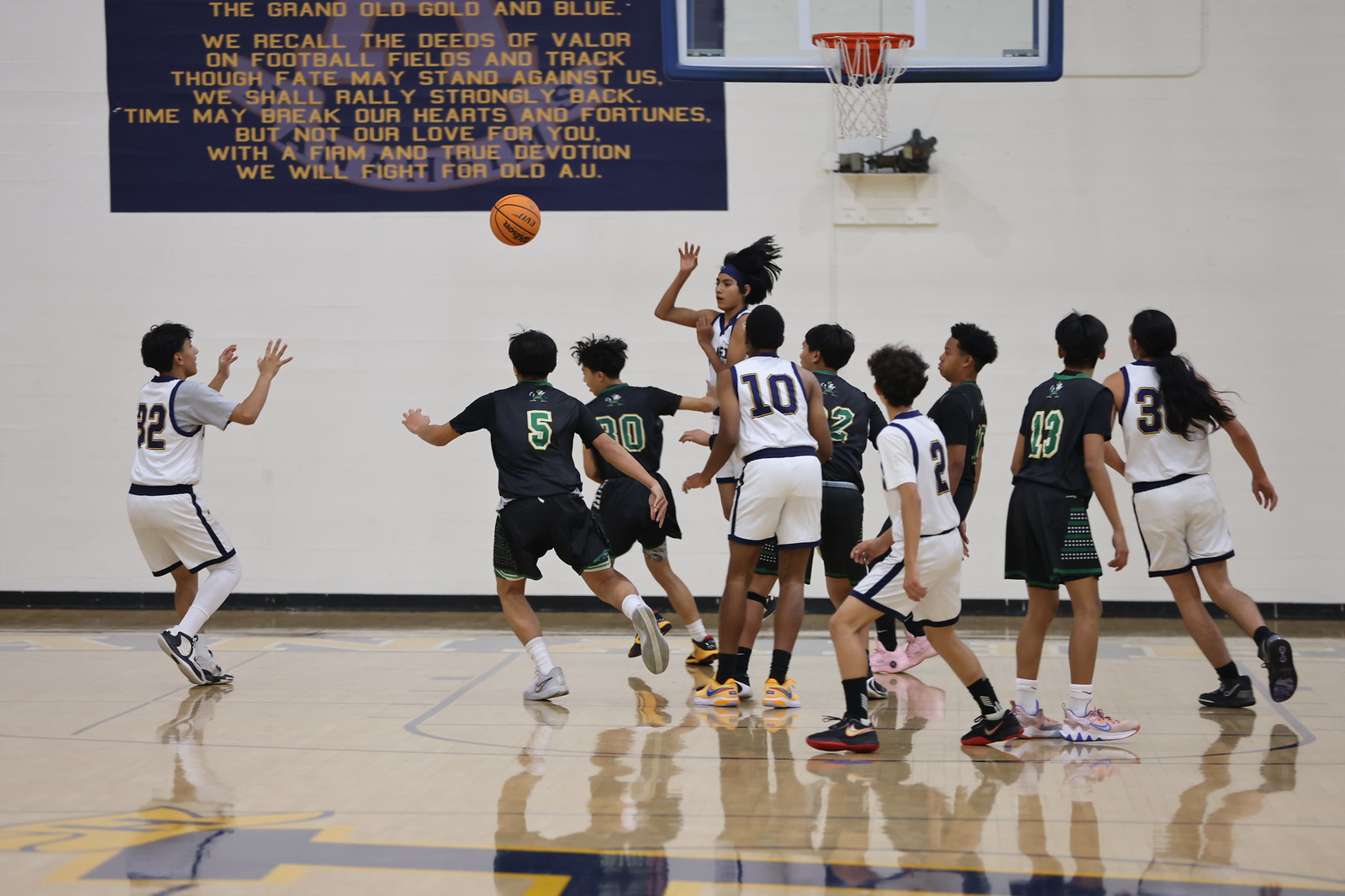The image captures an intense moment during a high school basketball game in a gymnasium, featuring what appears to be coed teams. The gym's white stone walls serve as the backdrop, adorned with a prominent blue and gold banner that reads, "The Grand Old Golden Blue. We recall the deeds of valor on football fields and track. Though fate may stand against us, we shall rally strongly back. Time may break our hearts and our fortunes, but not our love for you. With a firm and true devotion, we will fight for old A.U."

On the court, there are two teams: one in white uniforms with black stripes on their shorts, and the other in black uniforms with green numbers. The wooden floor is well-polished, marked with the traditional basketball lines. All eyes are on a player in a white uniform near the basket, who has just passed the ball out of the lane. The ball is directed towards a teammate in white, positioned about an eighth of the way from the left edge of the image. Meanwhile, players in black are reacting quickly, rushing towards the ball. The players are seen wearing a variety of shoe colors, including black, orange, and gray, adding a splash of color to the dynamic scene. The basketball hoop is mounted on the wall, indicating the game is taking place in a traditional gym setting. The vibrant energy of the game and the engaging atmosphere of the gymnasium are captured in this vivid photograph.